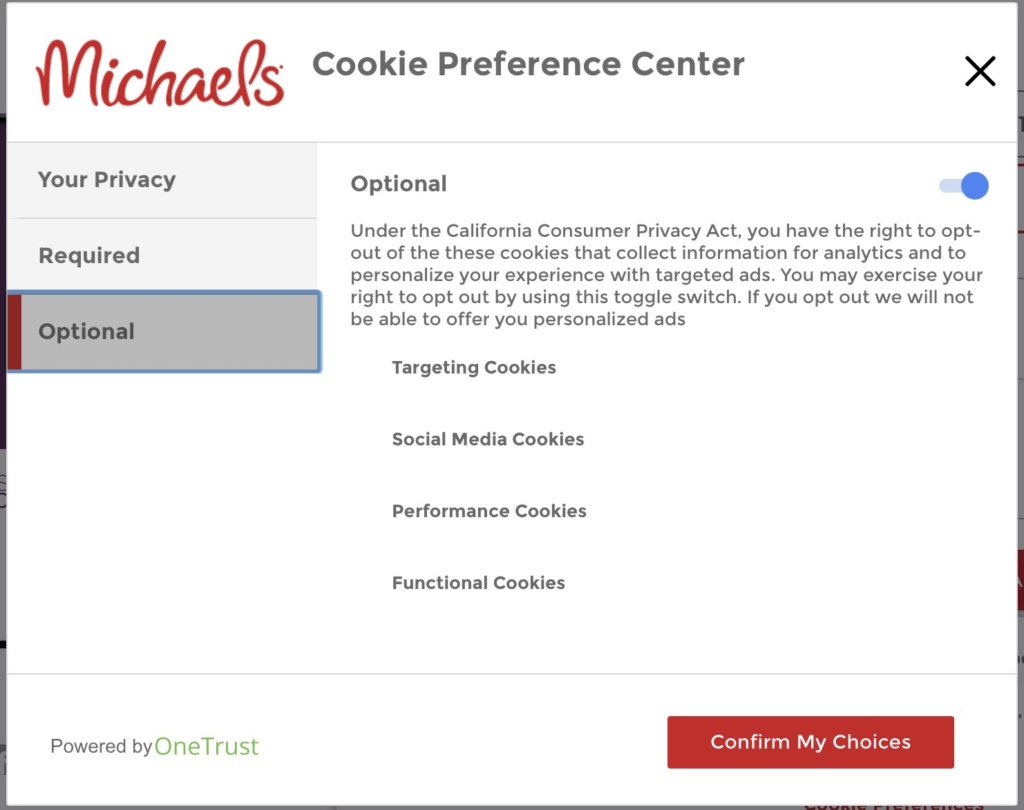Screenshot of the Cookie Preferences Center on the Michaels Website

The screenshot displays the cookie preferences interface on the Michaels website. The background is predominantly white. At the top left corner, the word "Michaels" is prominently displayed in red text. Adjacent to it, to the right in black text, it reads "Cookie Preference Center." On the top right corner of the interface, there is an option to close the window, indicated by an 'X'.

On the left sidebar of the screen, there are three distinct options listed in gray text:
1. Your Privacy
2. Required
3. Optional

The user has selected the "Optional" category. On the right side of the screen, next to the heading "Optional," there is a toggle switch, which has been toggled to the "on" position, indicated by its blue color. Below this section, there is a notice that states: "Under the California Consumer Privacy Act, you have the right to opt out of these cookies that collect information for analytics and to personalize your experience with targeted ads. You may exercise your right to opt out by using this toggle switch. If you opt out, we will not be able to offer you personalized ads."

Further down, four specific types of cookies are listed:
1. Targeting Cookies
2. Social Media Cookies
3. Performance Cookies
4. Functional Cookies

In the bottom left corner of the interface, the phrase "Powered by OneTrust" is presented, with "OneTrust" highlighted in green. On the bottom right, there is a red rectangular button with the text "Confirm My Choices" in white, allowing the user to save their cookie preferences.